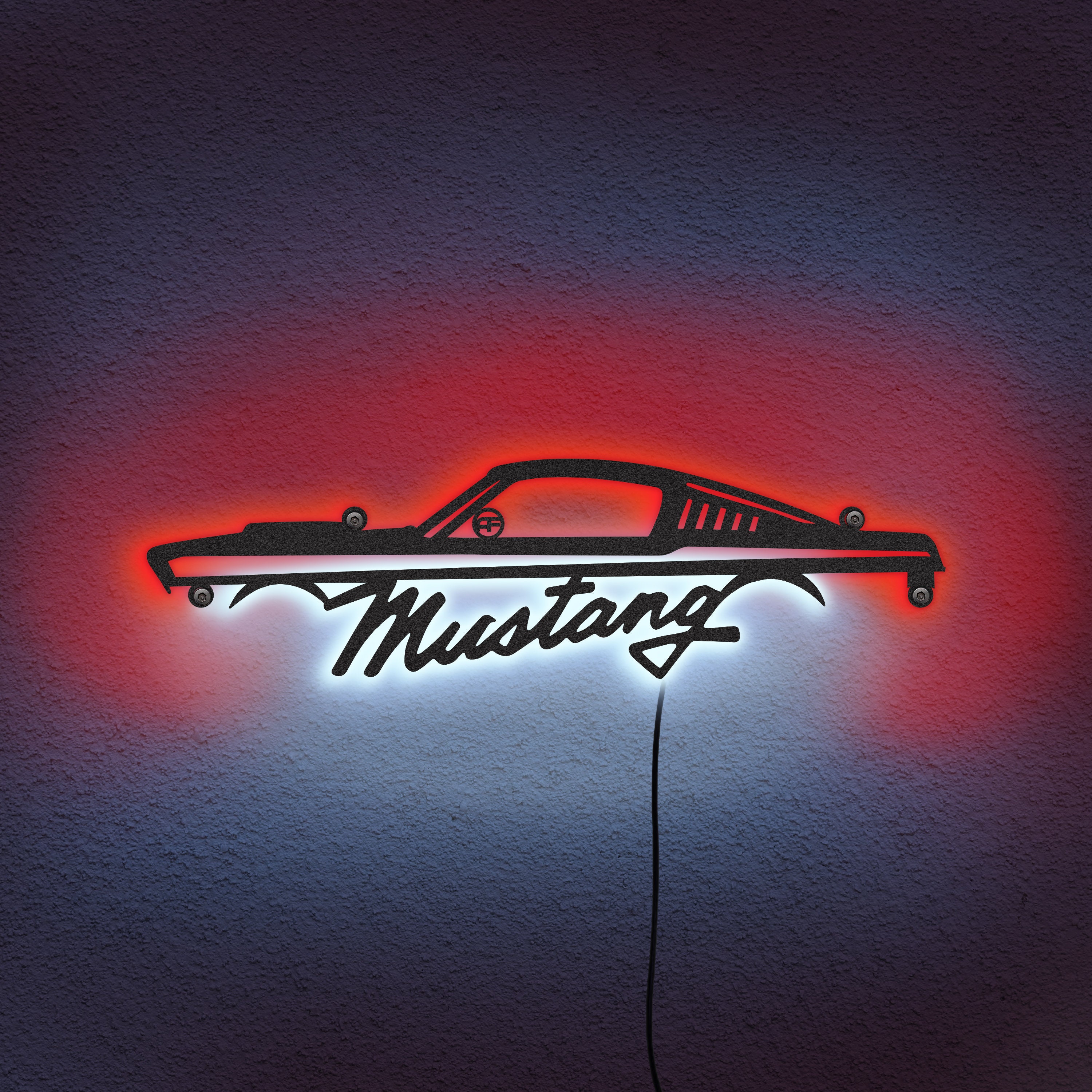The image depicts a decorative wall sign shaped like the dark silhouette of a car. The car appears to be a sleek sports model with an elongated body and an angled back passenger compartment featuring vented rear windows that taper to a point. Below the car silhouette, the word "Mustang" is crafted in a stylish, cursive typeface, seamlessly integrated into the design. The sign emits a red and white glow, casting a soft illumination on the surrounding area. A dark cord, visible against the white, textured wall, runs down from the sign, providing power and enhancing the overall aesthetic with a hint of industrial charm.